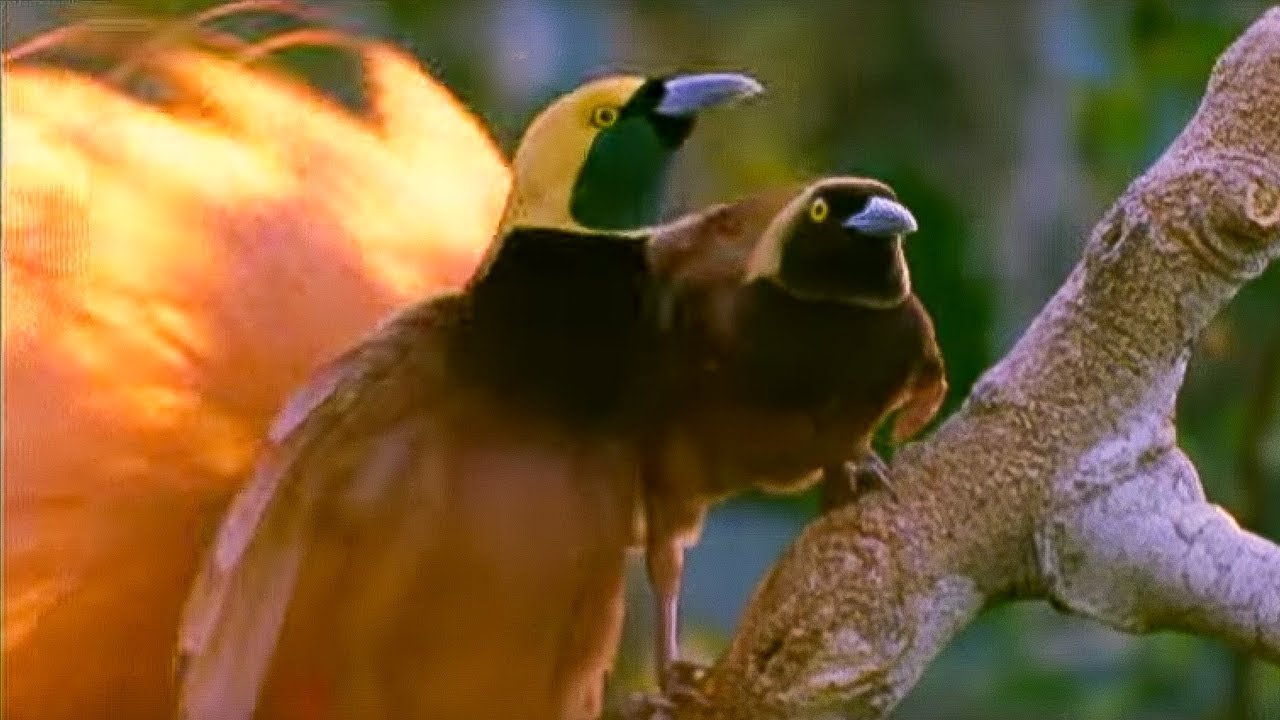The close-up image captures two birds perched side-by-side on a thick, light-colored, gnarled tree branch that cuts diagonally from the bottom center to the upper right of the frame. Despite the low resolution and slight blur, the birds' distinct features are noticeable. The bird on the left has a striking yellow head and neck, fading to a black upper body and brown towards its legs. It showcases a radiant plume of yellow-orange tail feathers that glows in the sunlight. Both birds possess small, gray beaks and bright yellow eyes. The bird on the right is primarily brown with yellow eyes and a gray beak, facing the camera while the bird on the left looks off to the right. The image appears to be a still frame from a video, evidenced by vertical distortions on the left side. This setting suggests a mating display, where the birds might be engaging in their side-to-side hopping dance.